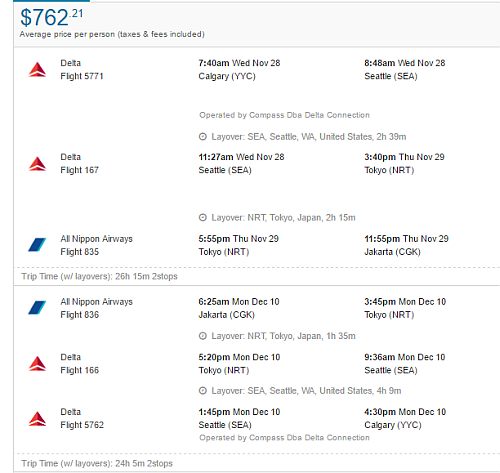**Detailed Caption:**

The image is dominated by a rectangular visual element with the right side incomplete, making it hard to determine the full length. Across the top, there's a gradient transition from teal to gray. Below this, a teal section features a dollar sign followed by the amount "$762.21". Underneath in black text, it reads "Average price per person (taxes and fees included)".

Beneath this section, a gray horizontal line extends across the width. Below the line, there's a series of flight details starting with Delta Airlines.

1. **Delta Flight 5771**     
   **Text:** The flight information is presented in alternating red and black text:  
   - "DELTA" in red   
   - "Delta Flight 5771" in black   
   - "7:40 AM WED" in black  
   - "November 28th | Calgary (YYC)" in black   
   - "8:48 AM WED | Seattle (SEA)" in black  
   - "Operated by Compass, DBA Delta Connection" in black    
   **Layover:**  
   - "Layover | Seattle, Washington, United States | 2H:39M"

2. **Delta Flight 167**  
   **Text:**  
   - "DELTA" in red   
   - "Delta Flight 167" in black   
   - "11:27 AM WED | November 28th | Seattle (SEA)" in black   
   - "3:40 PM THU, November 29th | Tokyo (NRT)" in black   
   - "All NIPPON Airways Flight 8.35" in black    
   **Layover:**  
   - "Layover | Tokyo, Japan (NRT) | 2H:15M"

3. **Connecting Flight:**  
   **Text:**  
   - "5:55 PM THU, November 29th | Tokyo (NRT)" in black  
   - "11:55 PM THU, November 29th | Jakarta (CGK)" in black

The caption meticulously describes the flight schedules, highlighting crucial points such as departure and arrival times, layover durations, and flight operators, offering a comprehensive summary of the itinerary.